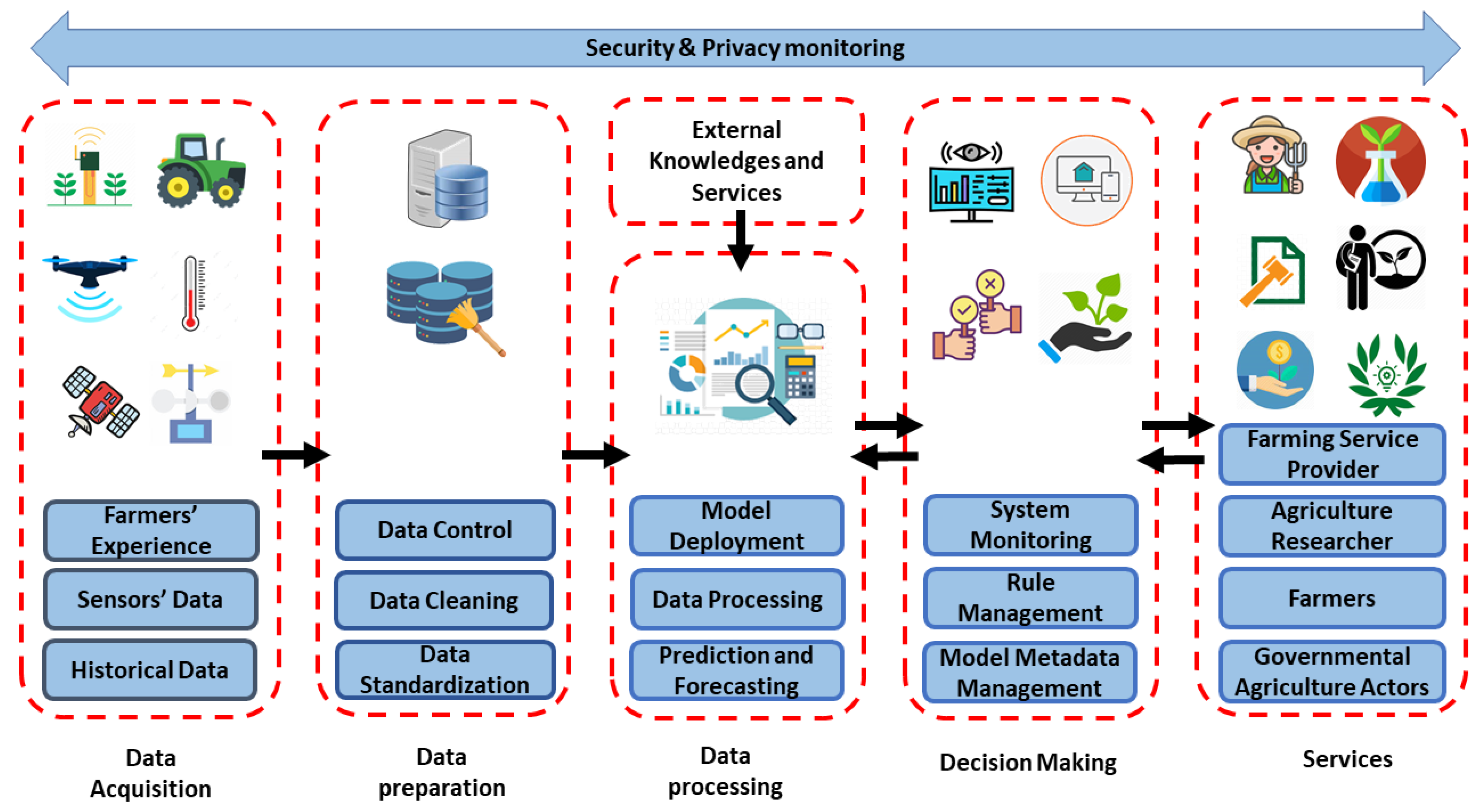The image is a meticulously hand-drawn infographic focusing on security and privacy monitoring within an agricultural context. At the top of the graphic, a light blue double-sided arrow spans its entire length, clearly labeled "Security and Privacy Monitoring." The infographic is organized into columns, each detailing a different stage of data management, indicated by red dashed lines and connected by black arrows.

On the far left, under the column labeled "Data Acquisition," the boxes depict various sources of agricultural data including farmer's experience, sensors data, and historical data. Visual elements include a tractor, plants, a thermometer, a satellite, and a wind indicator.

Next, moving right, the column "Data Preparation" shows a stack resembling gambling chips and is labeled with processes like data control, data cleaning, data standardization, and data preparation.

In the middle, the "Data Processing" column is labeled with tasks such as model deployment, data processing, predilection, and forecasting. It features images like a map with a magnifying glass, a pair of glasses, and a calculator.

To its right, the "Decision-Making" column highlights activities like system monitoring, rule management, and model metadata management. It includes icons such as two thumbs up (one with a checkmark, the other with an X), a hand holding a plant, a computer inside a circle, and a computer monitor with a Wi-Fi connection graphic.

The final column on the far right, labeled "Services," categorizes roles including farming service provider, agriculture researcher, farmers, and governmental agriculture actors. It is illustrated with a farmer, a plant, another person near a plant, a hand holding various objects, and a gavel.

The entire graphic features somewhat muted colors, primarily white and light blue, enriched with various other colors for additional details. The detailed and elaborate drawings suggest this could be a page from a manual or textbook, providing a comprehensive overview of technological advancements in farming, particularly focusing on data management and its significance in modern agriculture.